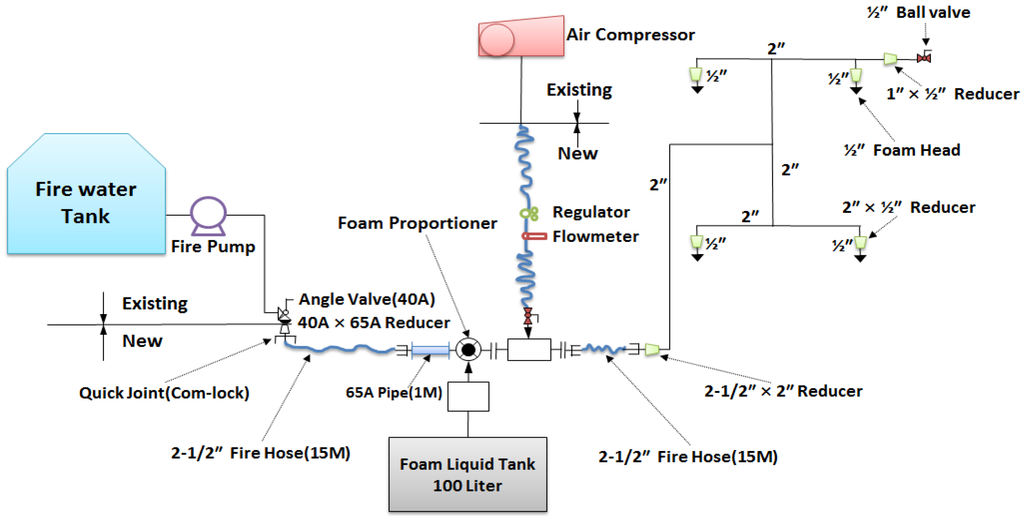The image is a detailed, horizontally oriented schematic diagram showcasing a fire suppression system. Dominantly black with black lettering, the central elements of the diagram include a variety of components, notably a pink gradient rhombus with a circle at the top middle labeled "air compressor". To the right of the air compressor, circles on the left side abut the word "existing," while the word "new" appears below, associated with horizontal and vertical arrows.

Key components in the diagram include a blue squiggly vertical line, three green balls labeled "regulator," and a pink rectangle marked "flow meter." A blue squiggly vertical line reappears beneath the flow meter. The arrangement continues with detailed parts such as a fire water tank colored blue, a fire pump, a gray foam liquid tank labeled "100 liters," and various other items labeled with sizes, inches, and amps.

On the left side, the fire water tank connects to a fire pump which leads to an angle valve marked "40A" and a quick joint labeled "comm lock," then proceeding to a fire hose. Subsequent components include multiple pipes, with another notable piece being the foam liquid tank at the bottom, directing flow into an interconnected system of boxes. Beneath these, labels such as "reducer valve," "two-inch hose," "ball valve reducer," and "foam head reducer," along with additional reducers, are depicted.

This comprehensive schematic illustrates the intricate connections and functionalities of a fire suppression system, encompassing the air compressor, fire water tank, foam liquid tank, and regulators, marked by an array of descriptive labels and vivid color coding for clarity.